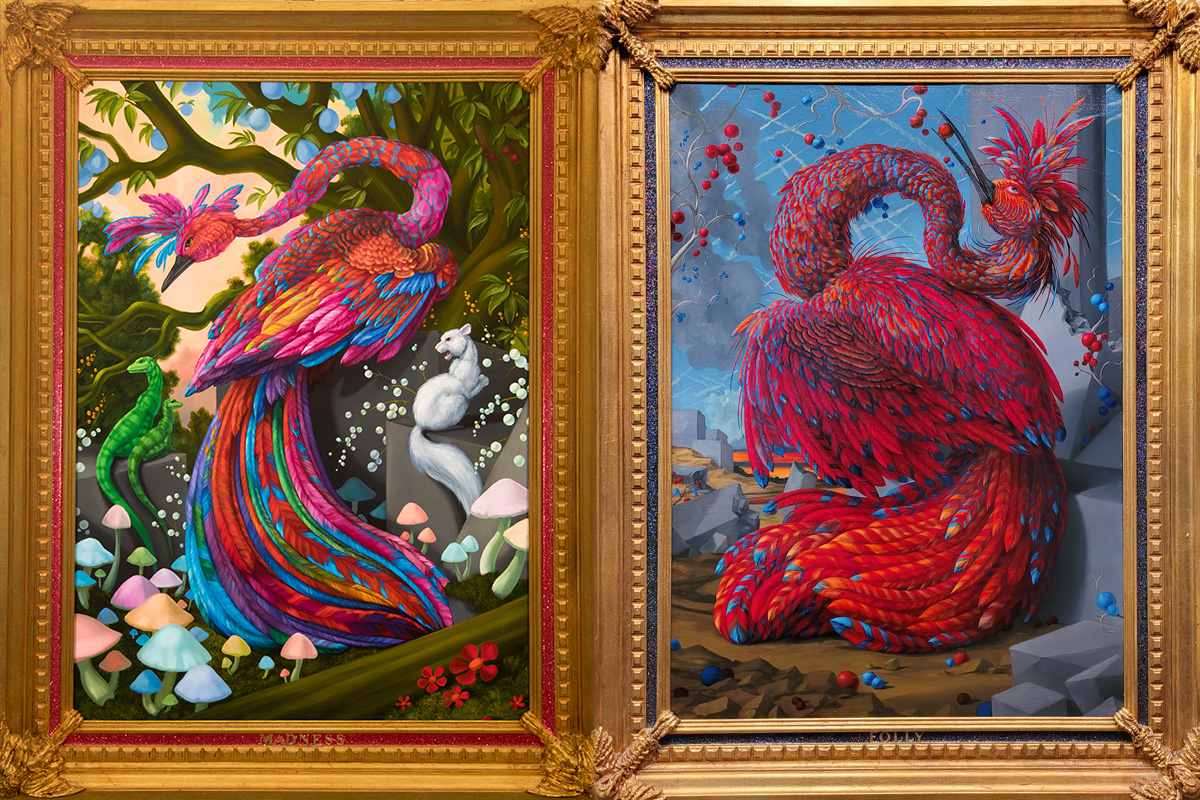The image features two side-by-side paintings, each framed in ornate gold with distinctively colored inner trims—pink for the left frame and blue for the right. The painting on the left showcases a fantastical bird resembling a peacock with radiant and diverse hues of pink, orange, yellow, green, and purple. The scene is vibrant with large trees in the background, adorned with blue fruits, and the ground scattered with multicolored mushrooms. Accompanying the bird are two green lizards and a small white creature that resembles a cat or squirrel with red eyes, all positioned on and around stone blocks.

Contrastingly, the right painting, bordered by a brighter gold frame with a blue trim, features a similar bird in an abstract form, marked by its curved neck and vivid red and blue plumage. This bird stands solitary in a more desolate environment, characterized by stone blocks and barren trees bearing red and blue fruits, devoid of other animals and the colorful surroundings seen in the left painting. Both artworks together create a vivid juxtaposition of lively, detailed habitat against a stark, more surreal setting.